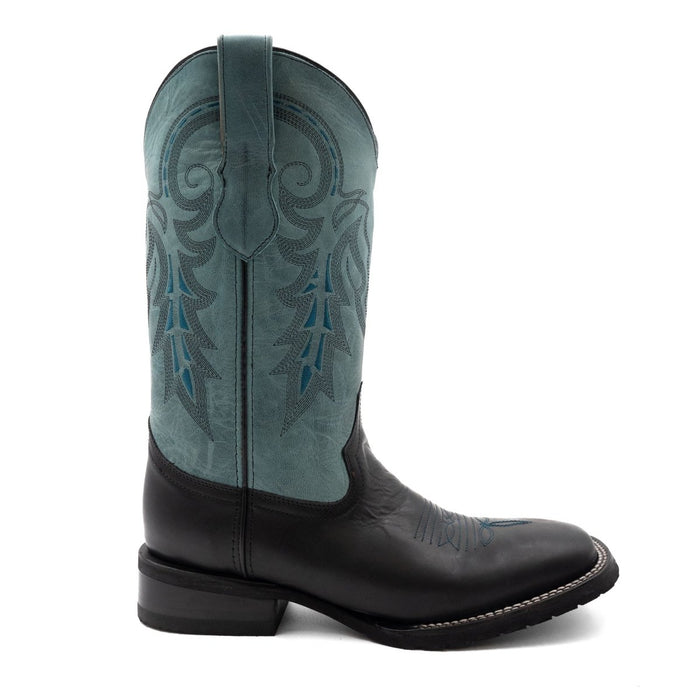This is a color photo of a single cowboy boot, positioned in right profile under soft, professional studio lighting. The boot features a two-toned design with a black leather lower section extending to the ankle and a turquoise to sky blue upper section that reaches calf height. The boot's upper section is adorned with intricate, embroidered stitching, showcasing a floral or leafy pattern reminiscent of William Morris designs, incorporating deeper blue detailing. The top of the boot is arched, following the shape of the decorative pattern, and includes a vertical strap for ease of pulling on. The sole is made of leather with a lug texture and is attached to the boot with white double stitching. The boot also features a thick heel and additional stitched detailing around the foot area. There is a shadow cast in the background, emphasizing the boot's detailed craftsmanship likely intended for promotional purposes.